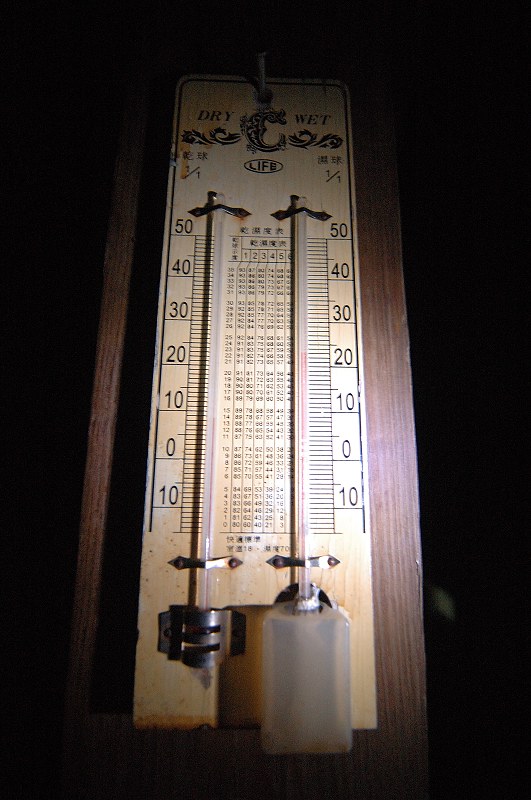This photograph features an intricate humidity and temperature tracker, reminiscent of a vintage thermometer. The device is divided into two sections labeled "Dry" and "Wet." At the top, ornate lettering encircles an elaborate "C", under which the word "Life" is inscribed. Decorative elements adorn each side of the "C" below the "Dry" and "Wet" labels.

Beneath each label, there are two thermometer-like gauges, both sharing the same scale ranging from 50 at the top to -15 at the bottom. The gauges are mounted on the wall with metal brackets at both the top and bottom. The bottom bracket on the left is notably thicker, providing additional support. On the right side, besides the metal brackets, there's a plastic jar attached below the "Wet" label, a feature absent on the "Dry" side.

Centrally located between the thermometers is a chart displaying various numbers and a selection of Asian characters at the top, suggesting additional information or calibration details related to the device's function. The entire setup appears to blend scientific instrumentation with artistic design, reflecting a blend of cultural and functional elegance.